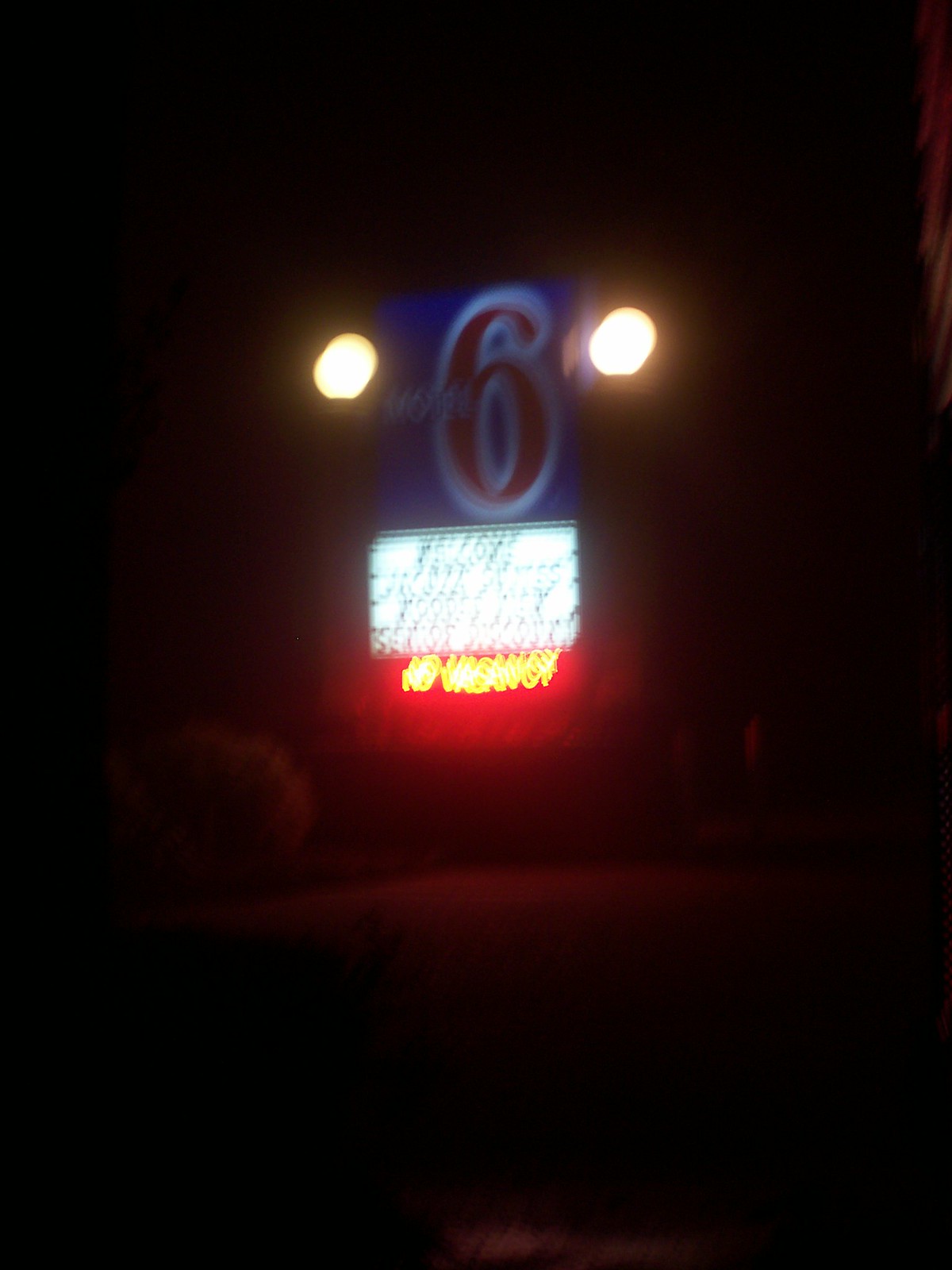The photograph captures a nighttime scene featuring an illuminated Motel 6 sign. The overall setting is enveloped in darkness, with the sky appearing completely black. The main sign, easily identified by the prominent Motel 6 logo, is a rectangular structure with a blue background and a large red "6" outlined in white. On either side of the sign are two white lights that enhance its visibility. Below the main logo, there's a smaller white sign that appears to offer additional information, although it's blurry and difficult to read. What stands out in red light is the "No Vacancy" sign, clearly indicating that the motel is fully booked. The left-hand side of the image shows some bushes, but their colors are indistinguishable due to the low light conditions. The photograph appears to be taken from across the street, providing a clear perspective of the illuminated sign amidst the dark surroundings.